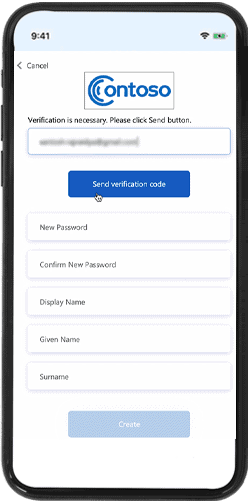A black electronic device, which could be a cell phone or tablet, is depicted with its side buttons clearly visible. The screen displays a white background with a light blue strip at the top. On this strip, the time "9:41" is shown on the left, and Wi-Fi and a green battery icon are on the right, suggesting it might be a tablet since there are no cell signal bars visible.

Directly below the strip, there are various interface elements on a white background. On the left side, a left arrow icon is visible beside a "Cancel" option. At the center of the screen, a grey-bordered, blue rectangle contains the text "conts tso" (presumably a corrupted or misinterpreted string).

The main message reads, "Verification is necessary. Please click the send button." Below this message is a blue "Send Verification Code" button, currently highlighted by a white hand cursor.

Further down, there are several input fields and corresponding labels: a thin rectangular box for a "New Password," another for "Confirm New Password," followed by fields for "Display Name," "Given Name," and "Surname." At the bottom center is a "Create" button, which appears grayed out, indicating that the fields have not been filled in and are necessary for activation.